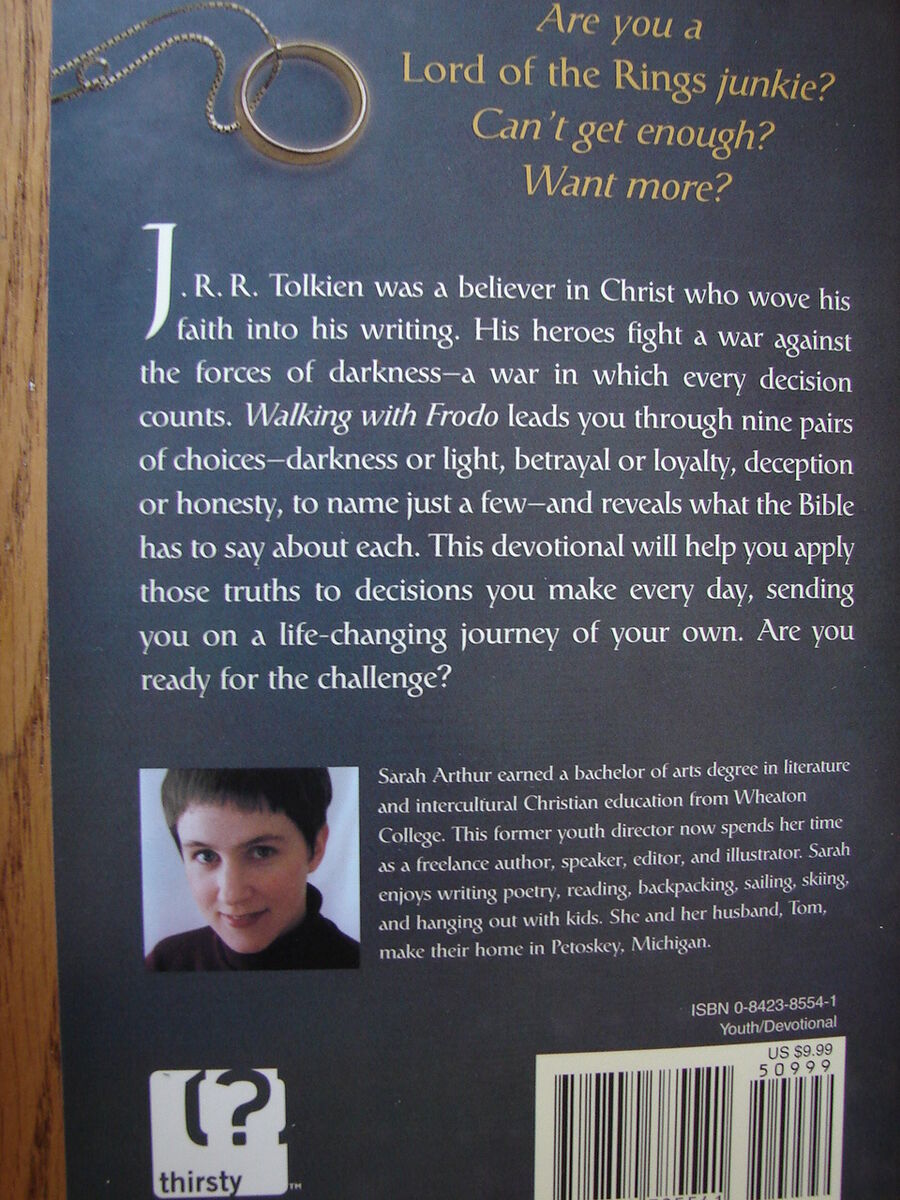This vertical rectangular image appears to be the back cover of a youth devotional book aimed at fans of the Lord of the Rings. The background is black with white text, bordered by a wooden brown edge on one side. At the top left, in golden text next to a brass ring hanging on a brass necklace, it asks, "Are you a Lord of the Rings junkie? Can't get enough? Want more?" This is followed by a white text paragraph that explains the book’s premise: J.R.R. Tolkien, a believer in Christ, interwove his faith into his stories. His heroes fought wars against darkness, with every decision carrying weight. The book works with Frodo’s journey, presenting nine pairs of choices—such as darkness or light, betrayal or loyalty, and deception or honesty—revealing what the Bible says about each. It aims to help readers apply these truths to their own lives, offering a life-changing journey and challenging the reader. 

Below this text is a small square image of Sarah Arthur, the author, who has short black or brown hair and is wearing a black turtleneck. Next to her photo, it describes her qualifications: She holds a Bachelor of Arts degree in literature and intercultural Christian education from Wheaton College and is a former youth director. Now, she is a freelance author, speaker, editor, and illustrator who enjoys poetry, reading, backpacking, sailing, skiing, and spending time with kids. She lives in Pensacay, Michigan, with her husband, Tom. At the bottom of the cover is a sales barcode with the price US $9.99, the number "50999," and the ISBN 0-8423-8554-1 Youth Devotional.